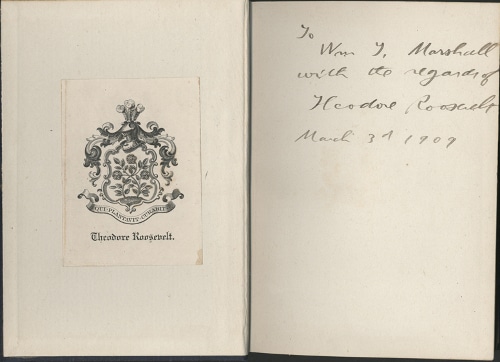The image depicts the open pages of a solid cardboard hardcover book with a tan cover. On the left page, there's a highly intricate black and white insignia featuring an extravagant crest decorated with a fleur-de-lis pattern and numerous flowers. At the bottom of the crest, there's a Latin banner with the name "Theodore Roosevelt" written in an old English type of font. The right page contains a handwritten note in cursive, which takes up less than half the page. The text is partially legible, mentioning "to T. Marshall with regards" and is signed by "Theodore Roosevelt." The note is dated March 31, 1909.